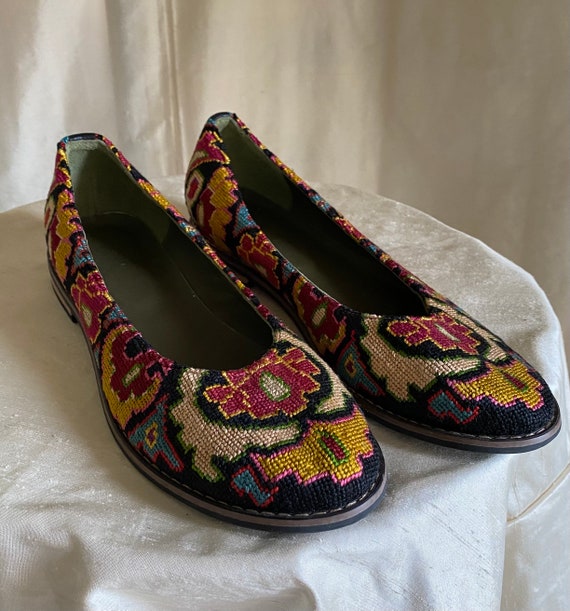The image is a detailed photograph of a vibrant pair of women's slip-on shoes, displayed on a small, round table or plinth, draped with off-white damask fabric featuring woven decorations. The shoes, which have narrow, rounded toes and gray linings, exhibit an intricate, hand-woven tapestry design reminiscent of a Turkish rug. Their colorful patterns include shades of red, yellow, pink, purple, blue, black, and green, with abstract geometric shapes and floral motifs adorning the fabric. The shoes' vibrant colors and striking patterns suggest they could be traditional or folk items, potentially showcased in a museum-like setting or highlighted for an online sale. The table and background are also covered in a light cream-colored fabric, and the shoes cast distinct shadows on the tablecloth.